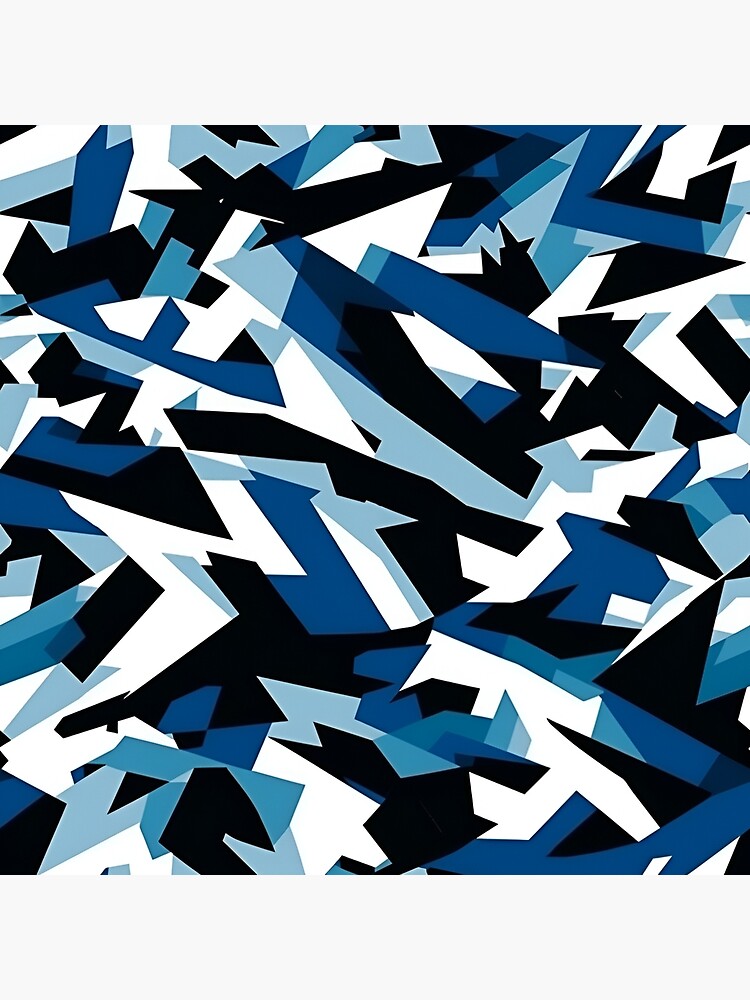The image depicts a vividly chaotic abstract composition characterized by jagged, angular shapes that evoke a sense of shattered glass or broken ice. The forms are difficult to identify, leaving room for interpretation as chevrons, chairs, lightning bolts, or even animals. Rendered in a striking palette of black, various shades of blue—including dark navy, light blue, and bright blue—and white, the pattern is complex and unstructured, with no clear background or singular recognizable object. The intricate geometric design appears almost animated, as if it were a zoomed-in sample of a larger print, and could function as dynamic phone wallpaper or an expressive wrapping paper print.